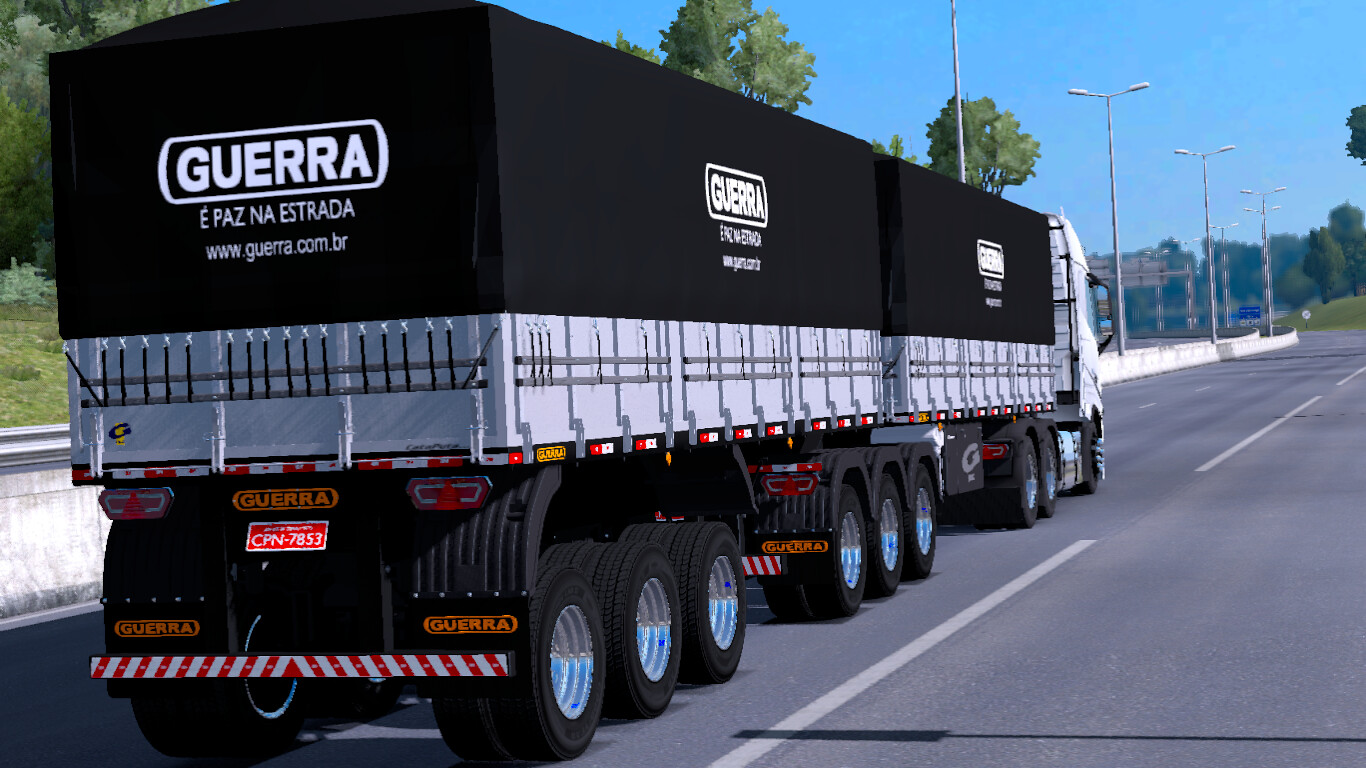The image appears to be an AI-generated, slightly pixelated scene resembling a computer game. It captures a sunlit day with a clear blue sky, featuring a large semi-truck traveling down a two-lane, rural highway. The perspective is from the rear right corner of the truck, revealing two massive silver containers on the truck bed, each wrapped in black coverings. Emblazoned in white, capital letters on the coverings is the word "GUERRA," enclosed in a white rectangle, with the additional Spanish phrase "Paz Na Estrada" below it. The truck, a massive 18-wheeler, has numerous wheels, likely up to 32 on the trailer alone, with the cab having two more. The scene is devoid of other vehicles, emphasizing the rural and tranquil nature of the setting. Concrete dividers line the road, punctuated by evenly spaced, unlit streetlights. Flanking the highway are subtle greenery and slightly sloping hills adorned with trees, further enhancing the serene environment.